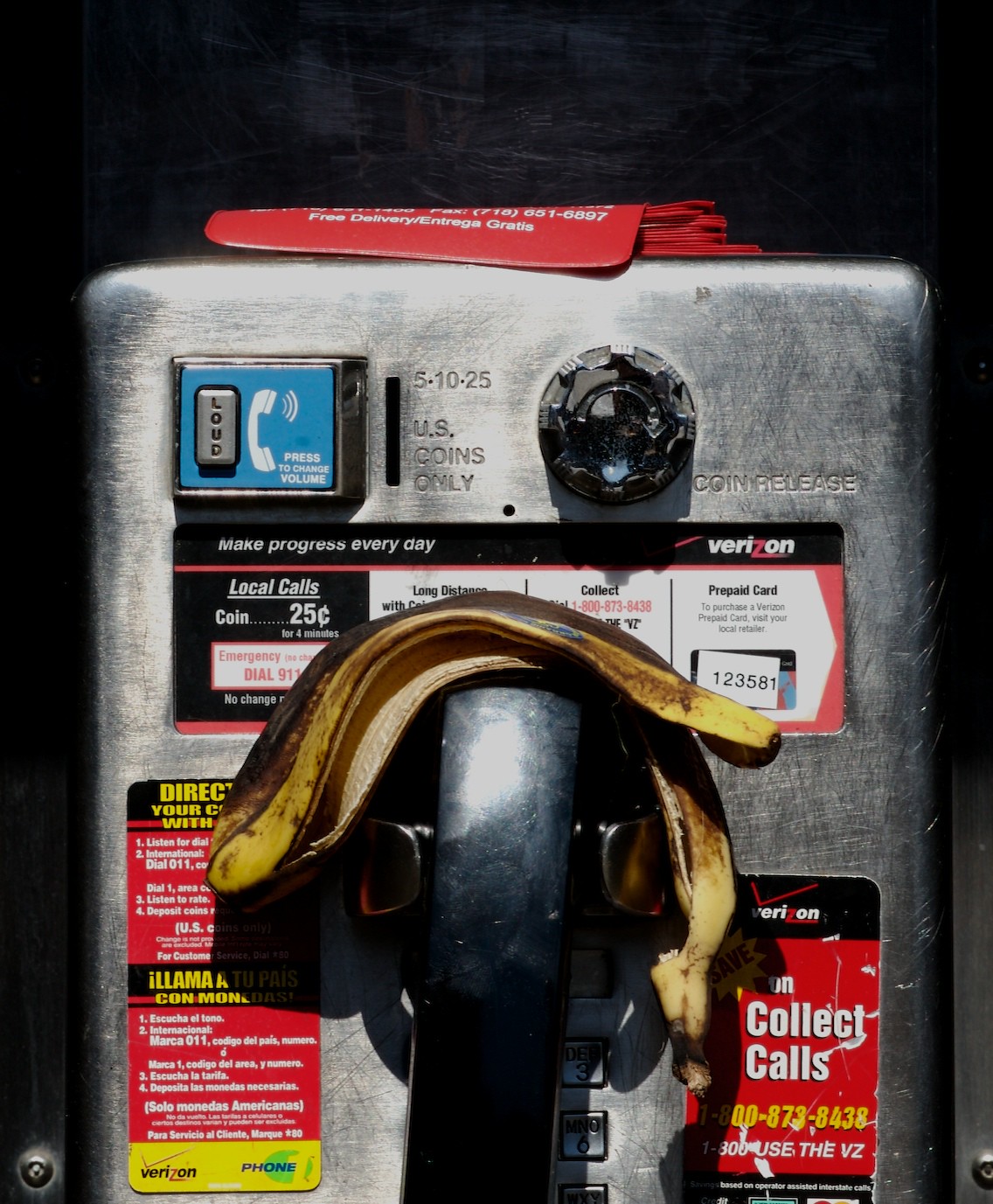This color photograph, captured in portrait orientation, features a detailed close-up view of an old-school payphone. The payphone, silver in color, is visible from about halfway down the keypad to the top. Dominating the scene is a black handset, securely placed in its cradle, with a yellow and brown banana peel draped over it. Various stickers and placards, some red and some not legible, adorn the payphone. Key features include a blue button at the top front labeled "press to change volume" and a black round knob with the engraving "coin release" on the top right. A vertical slot displays the denominations "5, 10, and 25 cents" along with the words "US coins only," and a horizontal sticker below provides information on making and placing calls. The payphone also displays references to Verizon collect calls and local calls for 25 cents. The payphone’s surface shows signs of wear, adding to the realism of the photographic representation.